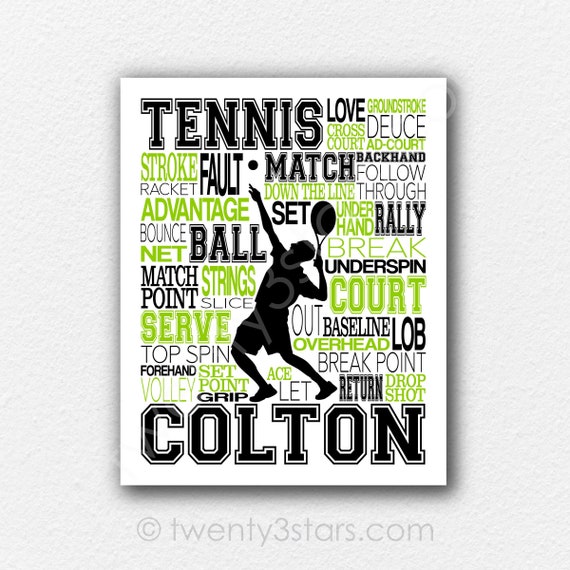The image is of a customized poster with a white background, designed for a person named Colton, as indicated by the large, black collegiate letters spelling "COLTON" at the bottom. Prominently displayed at the top left corner is the word "TENNIS" in black. The central focus of the poster is a black silhouette of a tennis player in mid-serve, with his right arm extended upwards tossing a ball, while his left arm wields a racket, poised to strike. The player's back is arched and his head is tilted upward, following the ball's trajectory. Surrounding this figure are numerous tennis-related words in varying sizes and fonts, both green and black, including "love," "ground stroke," "cross court," "deuce," "match," "backhand," "follow-through," "rally," "fault," "stroke," "racket," "advantage," "set," "bounce," "net," "match point," "strings," "court," "baseline," "lob," "serve," "slice," "top spin," "forehand," "grip," "volley," "add court," "down to the line," "underspin," "break," "out," "overhead," "break point," and "return." Below this dynamic collage is a gray background featuring a copyright notice indicating "20 number three stars dot com."